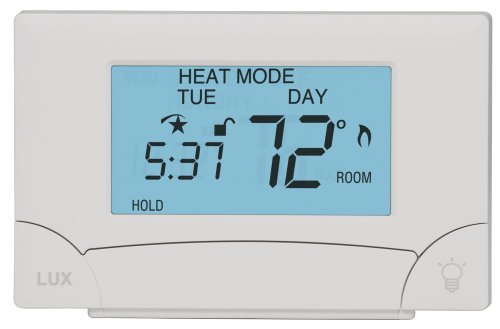The image displays a sophisticated thermostat, designed to control an air conditioning unit. The thermostat has a modern rectangular shape with elegantly rounded corners and is enveloped in a sleek gray plastic casing. Dominating the center is a light blue rectangular screen, which serves as the primary interface for the thermostat.

Prominently displayed in black letters on the screen is "HEAT MODE." Just beneath, the day of the week is indicated as "T-U-E," presumably Tuesday, flanked by a star-like icon with a curve at its top and an open lock symbol, indicative of an unlocked status. Below this section, the display indicates "537" followed by the word "HOLD."

On the right side of the screen, adjacent to the day indicator, the thermostat displays the current set temperature: "72°." Directly beneath this temperature reading, there is a small flame icon symbolizing heating mode, accompanied by the word "ROOM" below it.

The gray plastic casing features a distinct, curved design that elegantly transitions from left to right. In the lower left corner of the casing, the brand "LUX" is printed. Conversely, the lower right corner features a small light bulb icon, likely representing some form of illumination or additional feature.